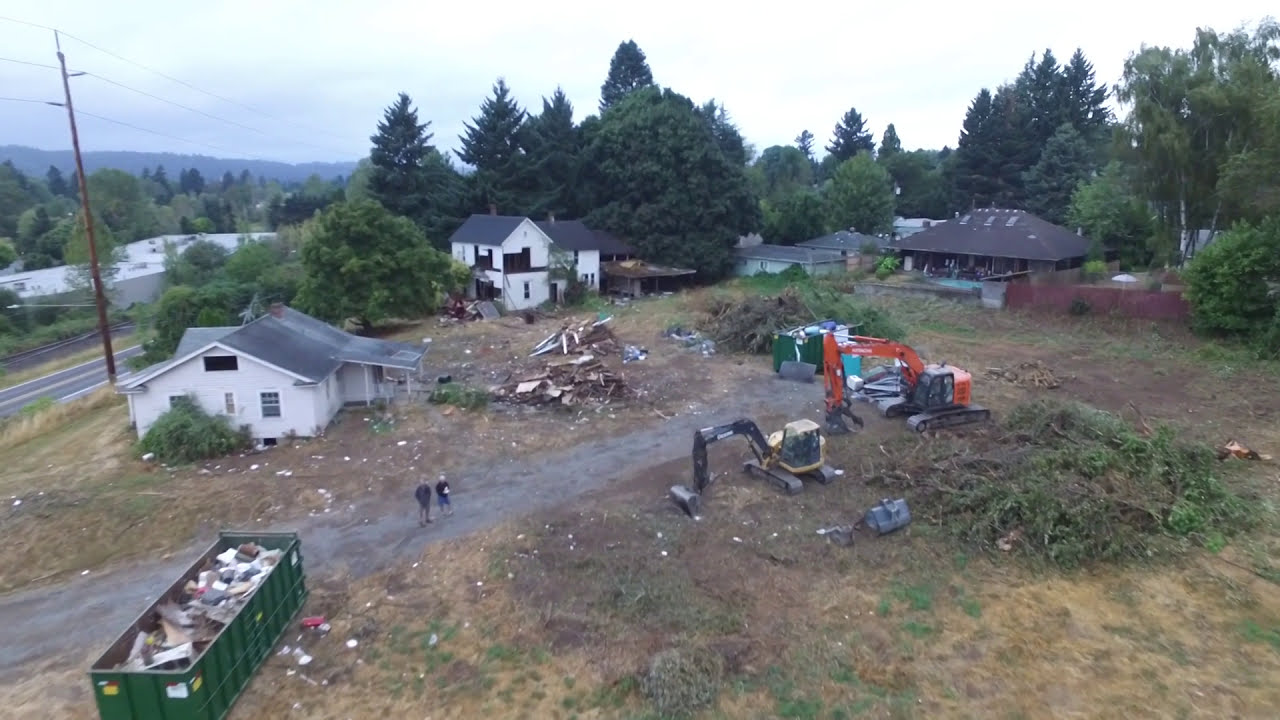The image depicts a rural area that appears to have been significantly affected by high winds or severe weather, possibly a storm. The scene is filled with debris, including construction materials and remnants of damaged structures, suggesting significant destruction. Central to the image, there are two excavating vehicles: an orange crane and a smaller yellow one, actively engaged in clearing the area. To the bottom left, a green dumpster brimming with garbage and remnants of buildings stands beside a dirt path where two people are observing the scene.

Scattered around the area, trees have been uprooted, and various construction materials are strewn across the grass, indicative of ongoing cleanup efforts. In the foreground, a demolished house's remains are piled up, while to its left, a complete white house with a black rooftop stands amidst the chaos. To the right, another white two-story house can be seen, with additional structures dotting the background.

The landscape is further characterized by a mix of tall pine and green trees, which frame the background along with distant mountains visible to the left. An old telephone pole and a road are noticeable on the left side of the image. The overhead perspective provides a comprehensive view of the entire scene, capturing the extent of the destruction and the ongoing efforts to restore the area.